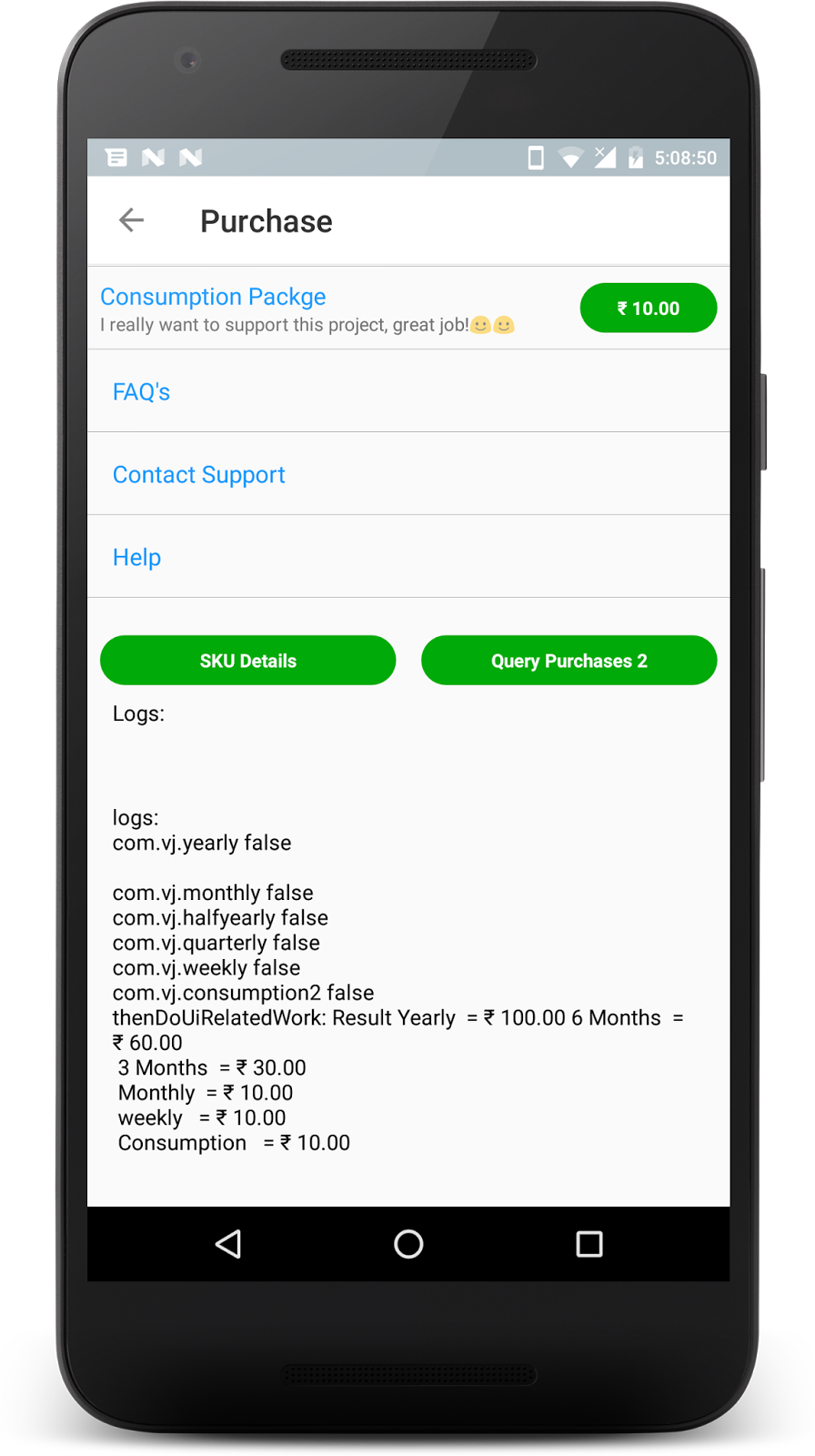In the image, there is a smartphone screen displaying a detailed interface related to a purchase transaction. The screen shows a left arrow icon, likely for navigation or going back. The battery icon features a thunderbolt symbol indicating it is currently charging, with the time displayed as 5:08:50 PM. 

Prominently, there is a blue section labeled "Consumption Package" related to the transaction details, reflecting a very supportive sentiment towards the project. The interface includes a green oval, underneath which "$10" is displayed next to a currency symbol. Additionally, there are options for "FAQs," "Contact Support," and "Help".

There are two green ovals on the screen. The first green oval, with white text, displays options like "SKU Details" and "Query Purchase." Below these, there is a list of log entries such as com.vj.yearlyfalse, com.vj.monthlyfalse, com.vj.halfyearlyfalse, com.vj.quarterlyfalse, com.vj.weeklyfalse, and com.vj.consumption2false. At the bottom, an incomplete line reads, "do U, Result Yearly equals," suggesting a partial programming script or data log entry.